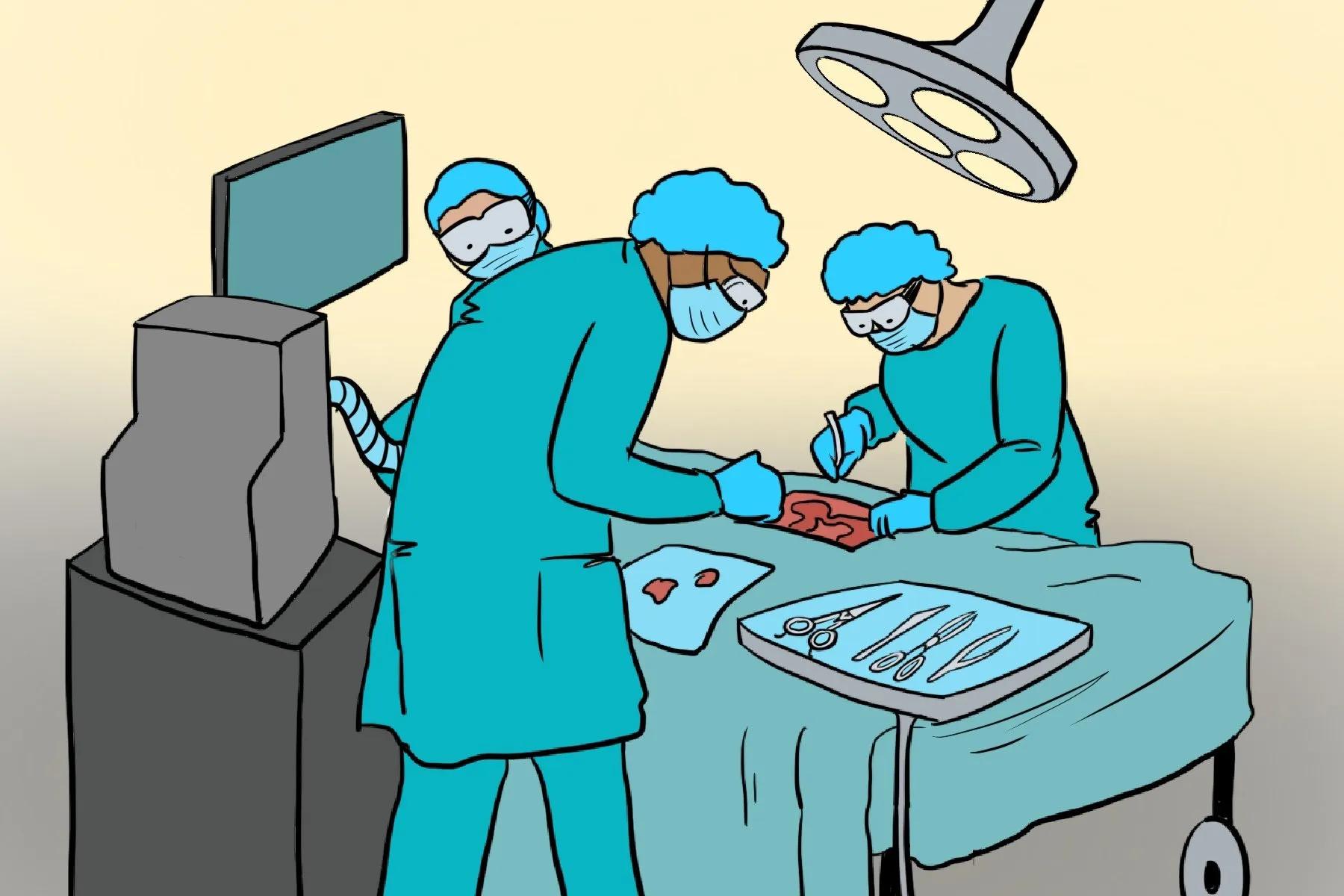This detailed cartoon-style drawing depicts a medical scene with three surgeons performing an operation. The background transitions from a light yellow to a light gray, creating a non-specific room-like atmosphere. At the center is an operating bed covered with a light green sheet, which has a cutout revealing shades of pink and red, hinting at exposed body parts in the abdominal area. The surgeons, comprised of two women and one man—two Caucasian women and an African American man—are clad in clean, white-blue scrubs that include a jacket and pants, along with blue caps, goggles, and face masks for full PPE. They appear busy and focused, with one woman holding a metal device, perhaps a surgical instrument, while nearby there is a tray of tools containing scissors, scalpels, and tweezers. Additional medical equipment is seen to the left of the surgeons, and a computer monitor is mounted on the wall, keeping track of the patient's vitals. The entire scene is designed in a style suitable for online publications or comics.